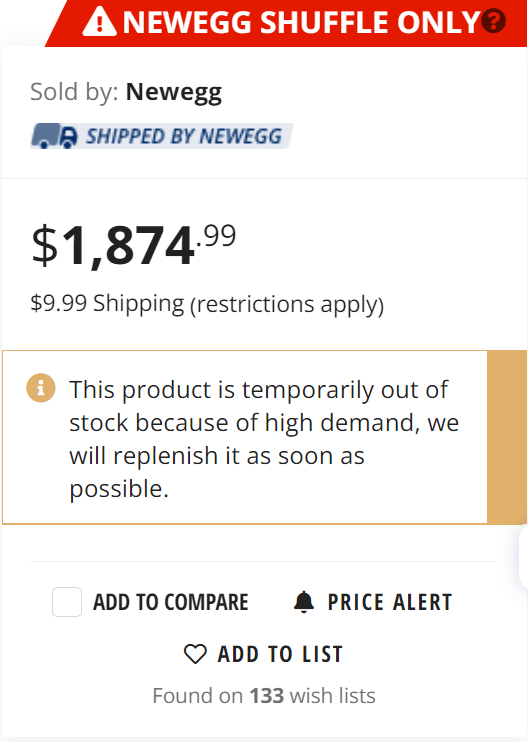A detailed screenshot taken from the mobile version of the Newegg website reveals the purchase attempt of a high-demand product, currently out of stock. The screenshot prominently displays a notification stating, “This product is temporarily out of stock because of high demand. We will replenish it as soon as possible.” The item’s price is listed at $1,874.99 plus shipping. 

At the top of the page, a distinctive bar reading “Newegg Shuffle Only” is visible, suggesting a restricted purchasing process for certain items. Further details indicate that the product is both sold and shipped by Newegg. Users are given multiple interactive options, including a toggle for product comparison, a price alert link, and an “add to list” button. Notably, the item is already found on 133 wish lists. The entire interface is set against a clean white background with black text, contributing to the overall clarity despite the array of information presented.

In essence, the screenshot captures the frustration of attempting to purchase a highly sought-after item that is temporarily unavailable due to its popularity.